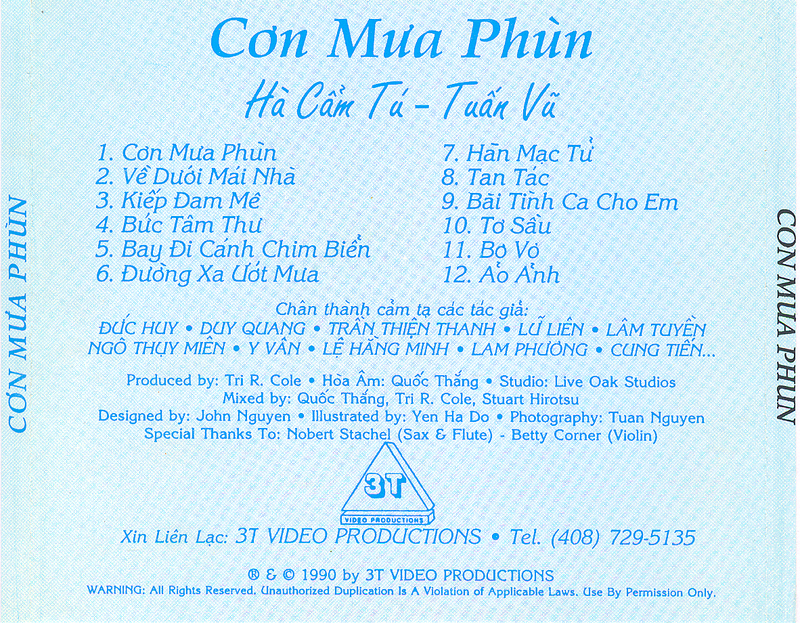This large square image, likely the back cover of a CD or musical album, features a subtle checked pattern on a sky blue background. Centered at the top in darker blue font are the words "Con Mua Phun," assumed to be the artist's name, followed by "Ha Com Tu - Tuan Vu," which appears to be the album title, both written in a non-English language. The album's tracklist is displayed in two columns: the left column numbered 1 through 6 and the right column numbered 7 through 12, each with names to the right of the numbers. Below the tracklist, in all caps white letters with bullet points separating each name, are additional credits. These include the production and mixing credits, including "Produced by Tri Arcol, Hoa Am Quoc Thang Studio, Live Oak Studios," and mixing credits for "Quoc Thang, Tri Arcol, Stewart Hiratsu." The design and illustration are credited to John Nguyen and Yen Ha Do, respectively, while photography is credited to Tuan Nguyen. Special thanks are given to Nobert Stachel of Saxon Flutes and Betty Corner Violin. Beneath these details is a triangular logo with three T's inside, representing 3T Video Productions, followed by their contact information, registered trademark, copyright from 1990, and a warning about unauthorized duplication. The final line states, "Xin Lin Locke, 3T Video Productions, telephone 408-729-5135," emphasizing the legal advisories regarding the album’s content.